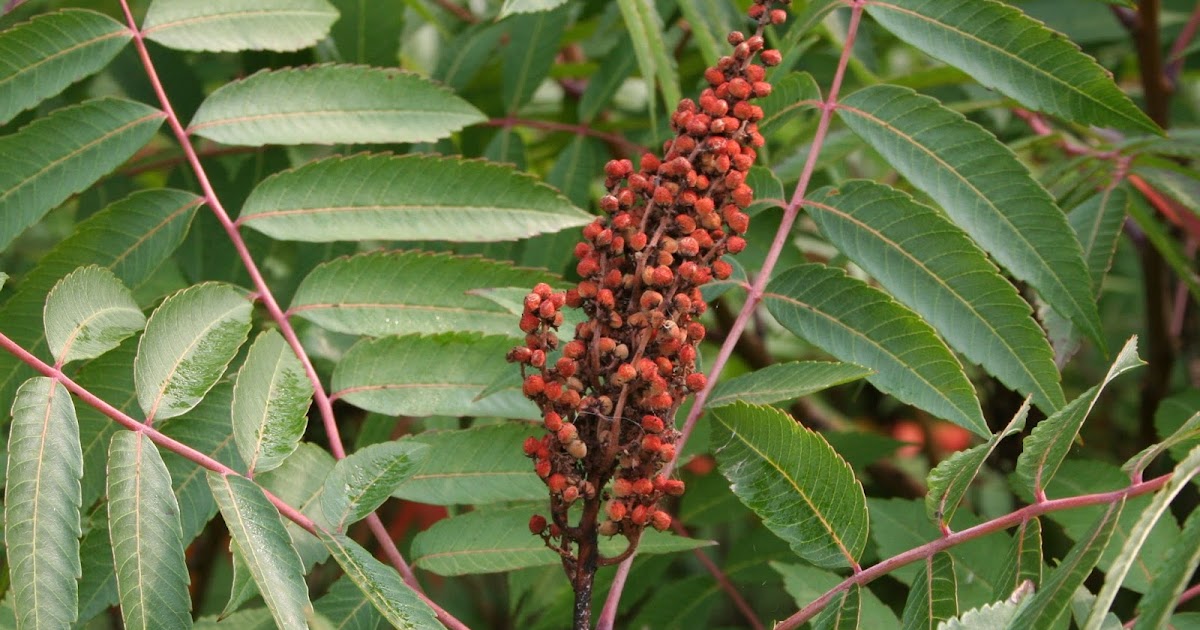This photograph captures a detailed, close-up view of a woodsy plant, specifically a type of sumac, either smooth or staghorn, from the genus Rhus. Central to the composition are clusters of vibrant red berries, which give the appearance of being rounded or bud-like, arranged along thin, extended branches that ascend toward the top right of the image. The central branch segments out into thinner, delicate branches covered in clusters of these red berries, with the terminal berries prominently positioned at the top edge of the photo. Flanking this central feature are long, narrow, serrated green leaves resembling palm fronds, although distinctly belonging to the sumac. These leaves are positioned opposite each other on the stems, contributing to a lush backdrop that envelops the entire scene. A faint stem can be seen descending towards the bottom of the frame, emphasizing the plant's intricate structure. The photo appears to be taken in bright light, with hints of dew or moisture adding a fresh, verdant quality to the foliage.